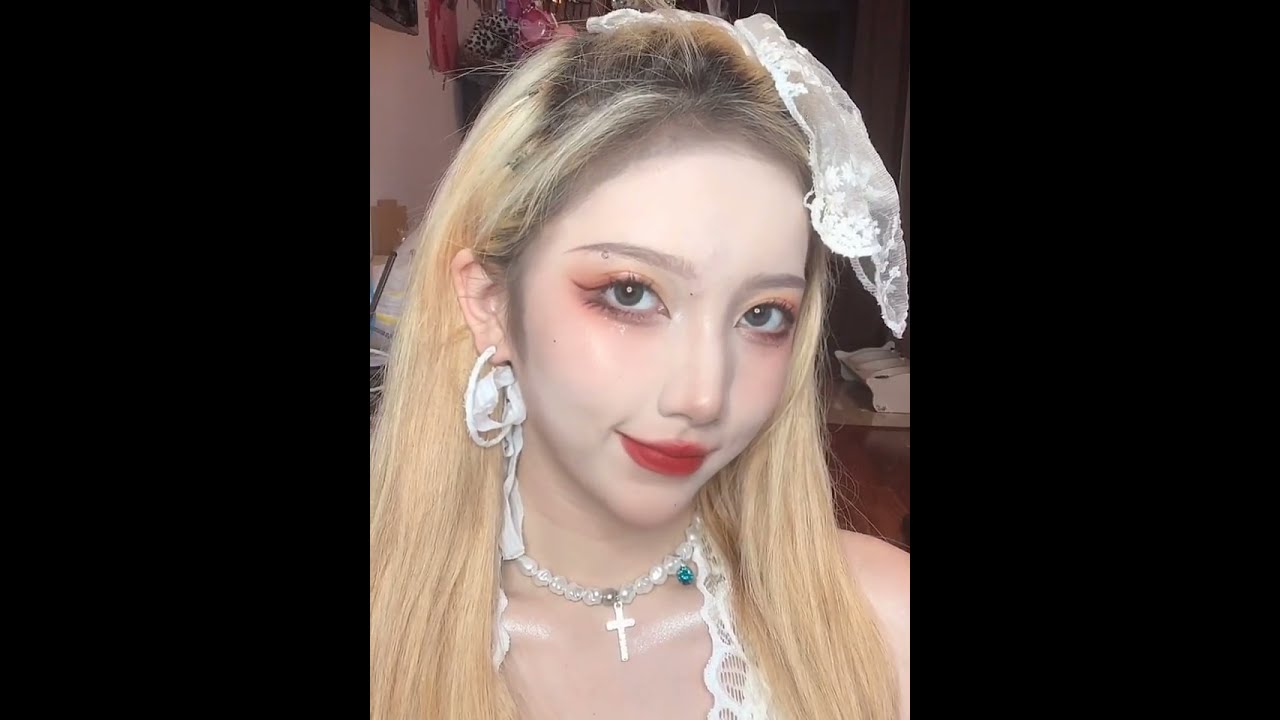A young woman, possibly in her late teens or early twenties, is posing for a portrait. Her head is slightly tilted to her left and she gazes directly at the camera with a faint smirk or smile. Her hair is predominantly blonde, with noticeable brown roots, and it is adorned with a delicate white lace ribbon, resembling a Madonna-esque style from the 80s. She has finely sculpted, frail features highlighted by heavy pink mascara and bright red lipstick. Her eyes are a striking greenish-blue, complementing her bold makeup.

She wears a white lace halter top, and around her neck is a beaded choker—mostly white beads, with one silver and one bright green bead, and a small silver cross pendant hanging from the center. She also has white hoop earrings visible on her right ear. The background features dated pink walls with pictures hanging on them, evoking a nostalgic feel. A desk cluttered with various objects is also visible, adding to the domestic atmosphere.

The image is bordered in black, framing the portrait in a way that draws attention to her detailed and distinctive appearance. Despite suggestions that she might be preparing for a wedding, the exact context remains ambiguous.